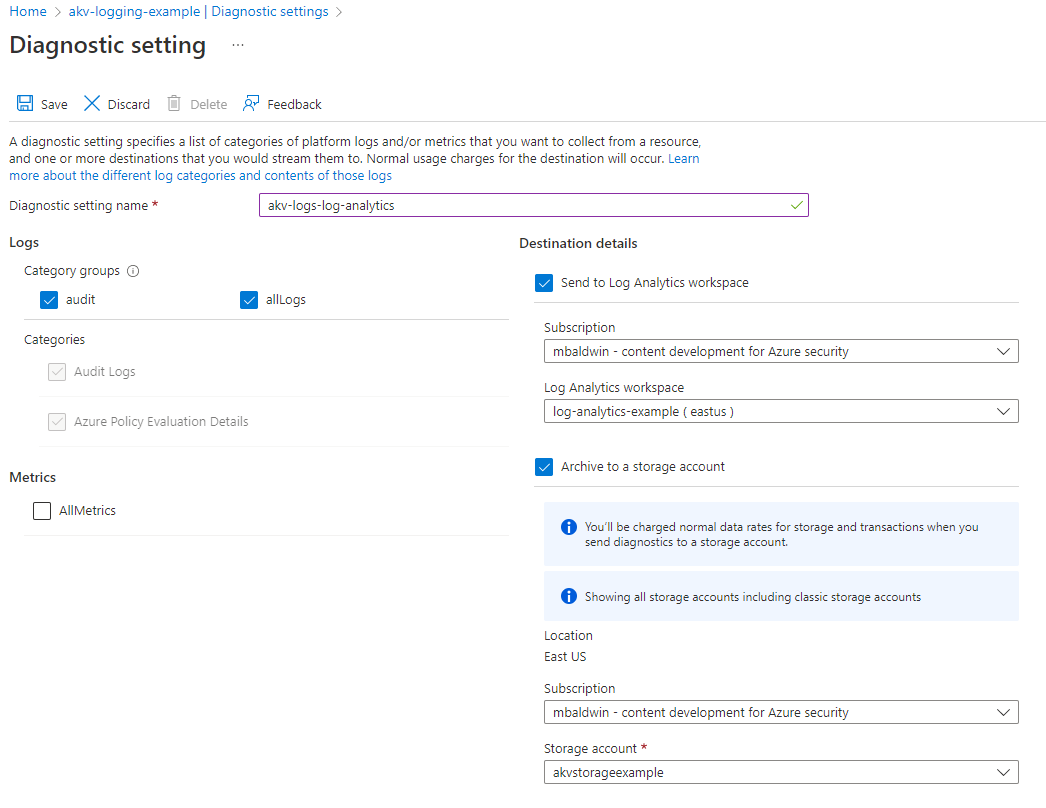Home Screen - AKV Logging Example: Diagnostic Settings Overview

The screenshot displays the "Home" section of the AKV Logging Example under Diagnostic Settings. At the top, several options are visible: "Save," "Discard," "Delete" (although "Delete" is not selectable), and "Feedback."

The Diagnostic Setting page outlines the following functionalities:
- Specifies categories of platform logs/metrics to collect from a resource.
- Configures one or more destinations for streamlining these logs/metrics. Note that normal usage charges apply for the specified destinations.
- A "Learn More" option is available to get details on different log categories and log contents.

Beneath this, the section "Diagnostic Setting Names" is labeled with an asterisk, indicating it is a required field. An open input field shows "AKV Logs Log Analytics." 

The layout divides into two main columns: "Logs" on the left and "Destination Details" on the right.

- First, under "Category Groups," there are options for "Audit" and "All Logs."
- The setting option "Send to Logs Analytic Workspace" indicates its selection.

Further details include:
1. **Subscription**: A drop-down menu shows "mBaldwin, Content Development for Azure Activity."
2. **Log Analytics Workspace**: Another drop-down menu lists "Log Analytics Example, ETAS, or EASTAS."
3. **Archive to Storage Account**: This feature is checked and notes standard data rate charges. It also indicates that all storage accounts, including classic ones, are shown.
   - The location is specified as "East US," with additional storage account examples provided in drop-down menus.

This detailed descriptive caption captures all essential elements and functionalities presented in the screenshot, providing clarity on the diagnostic settings and configuration options available.